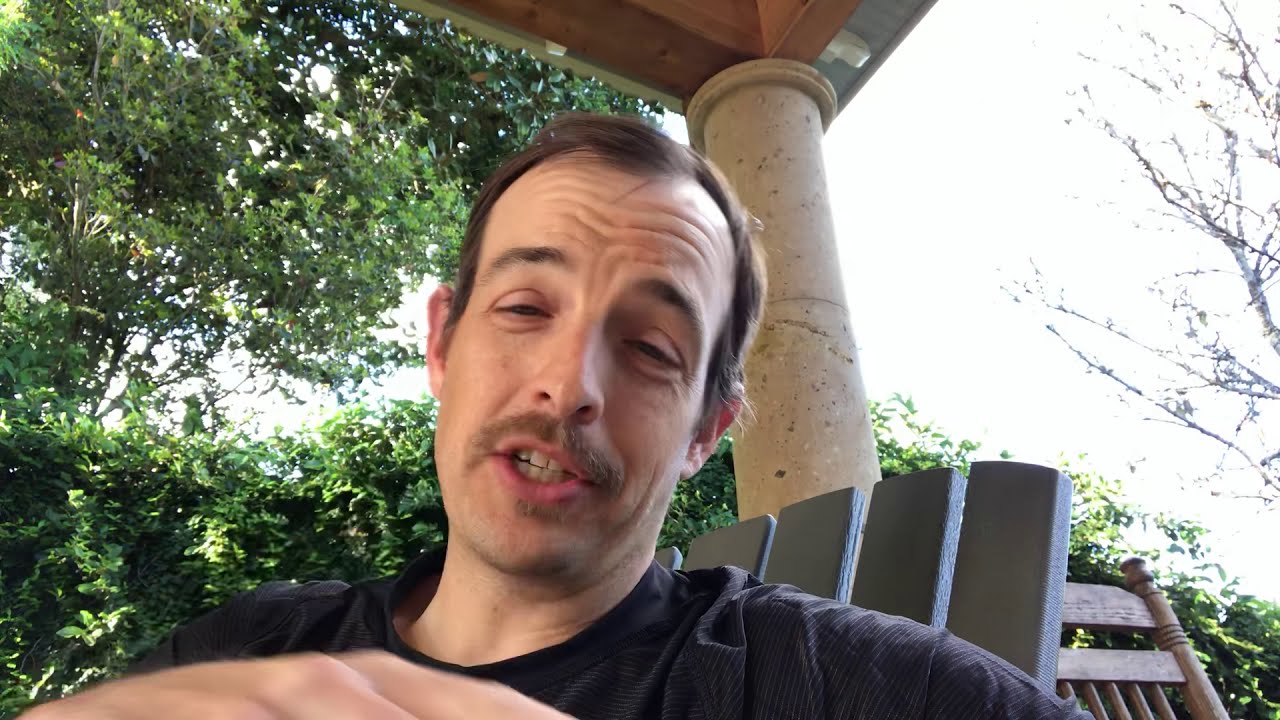The photograph portrays a middle-aged white man, likely in his 40s, with short, balding brown hair and a brown mustache. His head is centered in the wide, rectangular frame, slightly tilted to the right as he looks directly at the camera with a partially open mouth, as though he is speaking. His eyes appear somewhat baggy and semi-closed, and his forehead has visible wrinkles, emphasizing his expressive demeanor.

He is dressed in what seems to be a black t-shirt, possibly adorned with thin white stripes. The man is seated on a gray wooden chair with slats, while another brown wooden chair is positioned behind him to the right.

The setting suggests an outdoor location, likely a covered porch or terrace. Behind the man to his right is a cement cylinder supporting a brown awning or roof structure. The background features a mix of greenery, including tall green hedges, leafy trees to the left, and bare branches on the right, hinting at a garden or front yard environment. The overall impression is of a casual and candid moment, possibly a still from a vlog or broadcast.